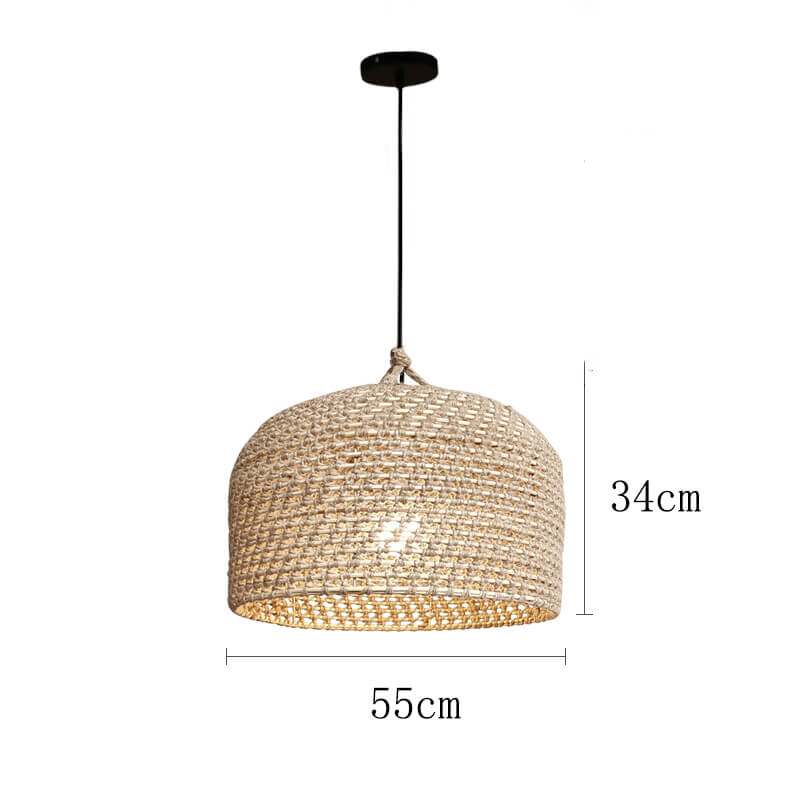This image depicts a highly detailed product photo of a unique Heng light. The lamp features a single bulb encased in an intricately woven, tan-colored shade that takes on the appearance of an upside-down basket. The materials used in the weaving could be wicker, wool, or bamboo, adding a rustic, handcrafted appeal. The lampshade measures 34 cm in height and 55 cm in width, not including the supporting elements. A sleek, black metal pole extends from a black circular disc attached to the ceiling, supporting the lamp's entire structure. Set against a plain white background, the photo highlights the lamp's craftsmanship and design, indicating it may be intended for sale, possibly as part of a display case or an art piece suitable for home decor.